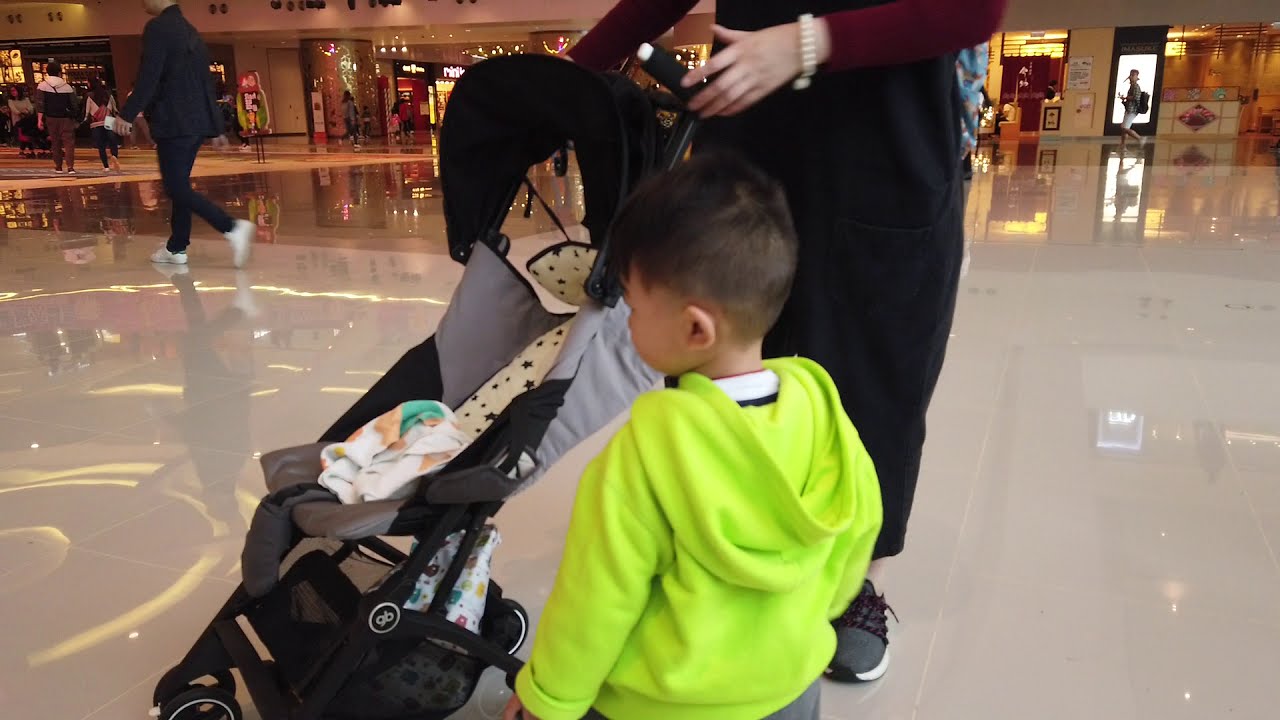In the image, a young boy is seen walking beside a black baby stroller, which is being pushed by his mother in a bustling shopping mall. The child, who has thin brown hair styled in a short crew cut, is wearing a bright neon green hoodie with a white shirt peeking through the collar. He appears to be looking away to the left. The stroller is notable for its black frame and the presence of a small white blanket or towel neatly wrapped in the seating area, but it does not hold a baby. The mother, only the bottom half of whom is visible, is dressed in black pants, black shoes, and a red shirt, with a distinctive white pearl bracelet on her wrist. Her right hand is positioned behind the stroller, while her left hand appears to be reaching towards the handle. In the back left corner of the image, another person dressed in black with white shoes is walking away. Further in the background, a man in a black jacket with a white top half and red pants, and a woman in a white shirt and black pants, are seen walking towards the top left corner. The shiny, glossy floor of the mall reflects the light from chandelier fixtures above, and the background is filled with various store entrances adorned with large, illuminated displays and logos.